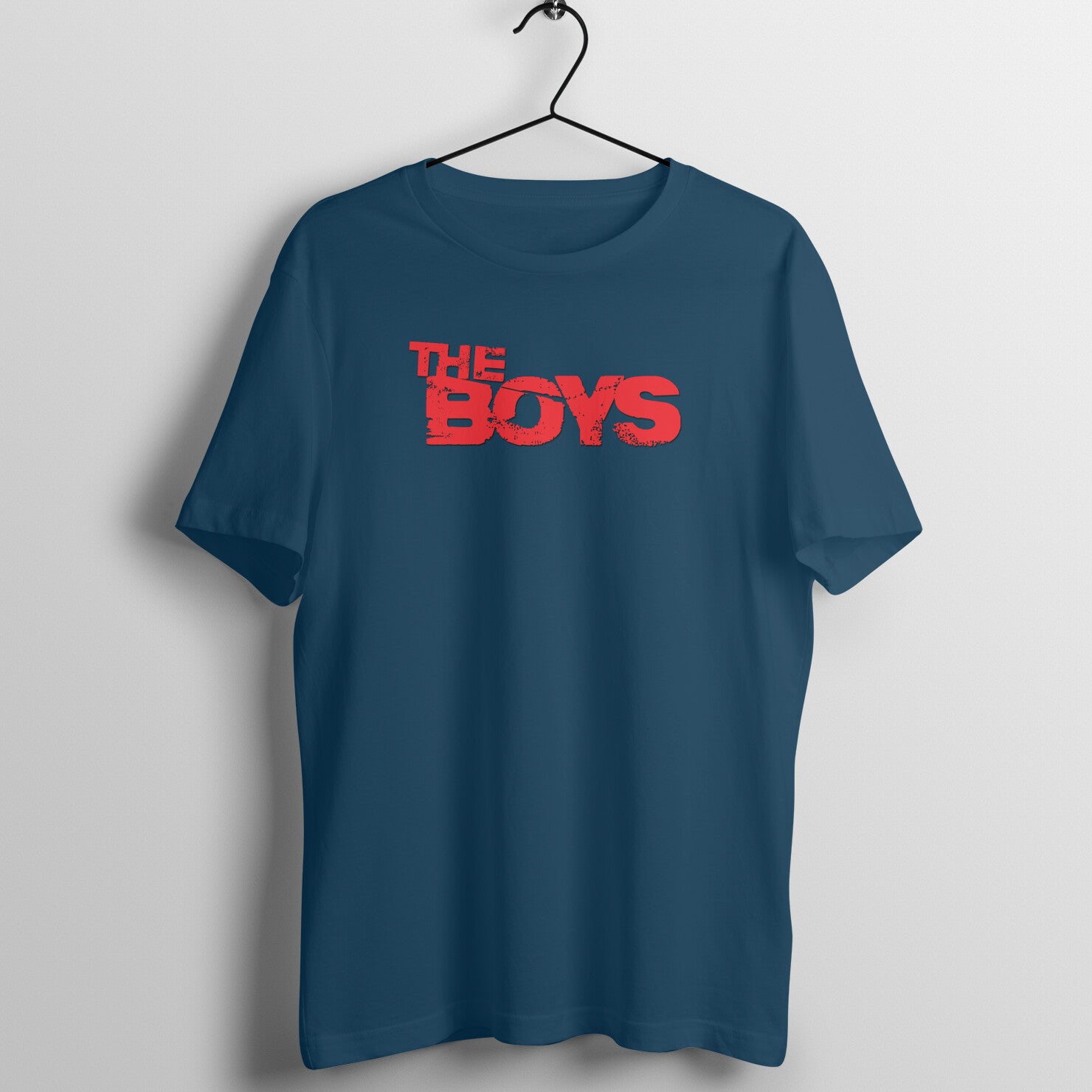This image features a navy blue T-shirt hanging on a black coat hanger, which is suspended from a small silver hook attached to an off-white wall. The shirt, likely a size small or medium, displays "THE BOYS" in large, distressed red letters, reminiscent of spray paint, across the front. The design appears slightly rippled due to the way the shirt is hanging. The black hanger casting shadows to the bottom and left side accentuates the textured look of the garment. The T-shirt seems to be promoting the Amazon Prime show "The Boys" and might be sold through various channels, possibly including fan-made outlets like Etsy or official retailers such as Amazon. The shirt's simple, stitched trim on the sleeves and bottom emphasizes its casual, everyday wear appeal.